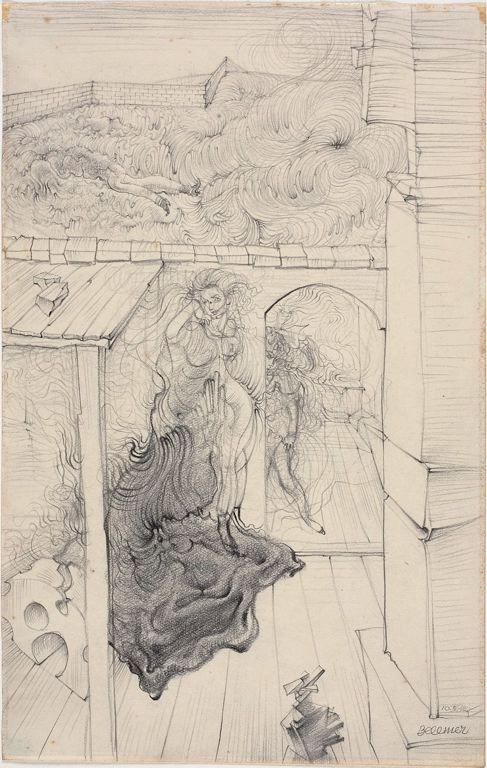The image is an elaborate black ink pen sketch depicting a young maiden scantily dressed in flowing, sheer material, standing within an open passageway of a building. The central figure, the woman, is positioned on a wooden floor with a wooden roof patio to her left. Behind her is a wall with a cut-out passageway. To her right is a large wooden structure, possibly a column, and further beyond that, a grassy field enclosed by a fence. The background features a mixture of brickwork and hay, resembling a barn-like setting. The black and white sketch also includes details such as a couch on the left and possibly a tool in the foreground. The scene conveys a sense of an interior space, potentially a brothel, with women coming in and out of a doorway. The artwork is signed at the bottom right-hand corner, though the signature is indistinct.